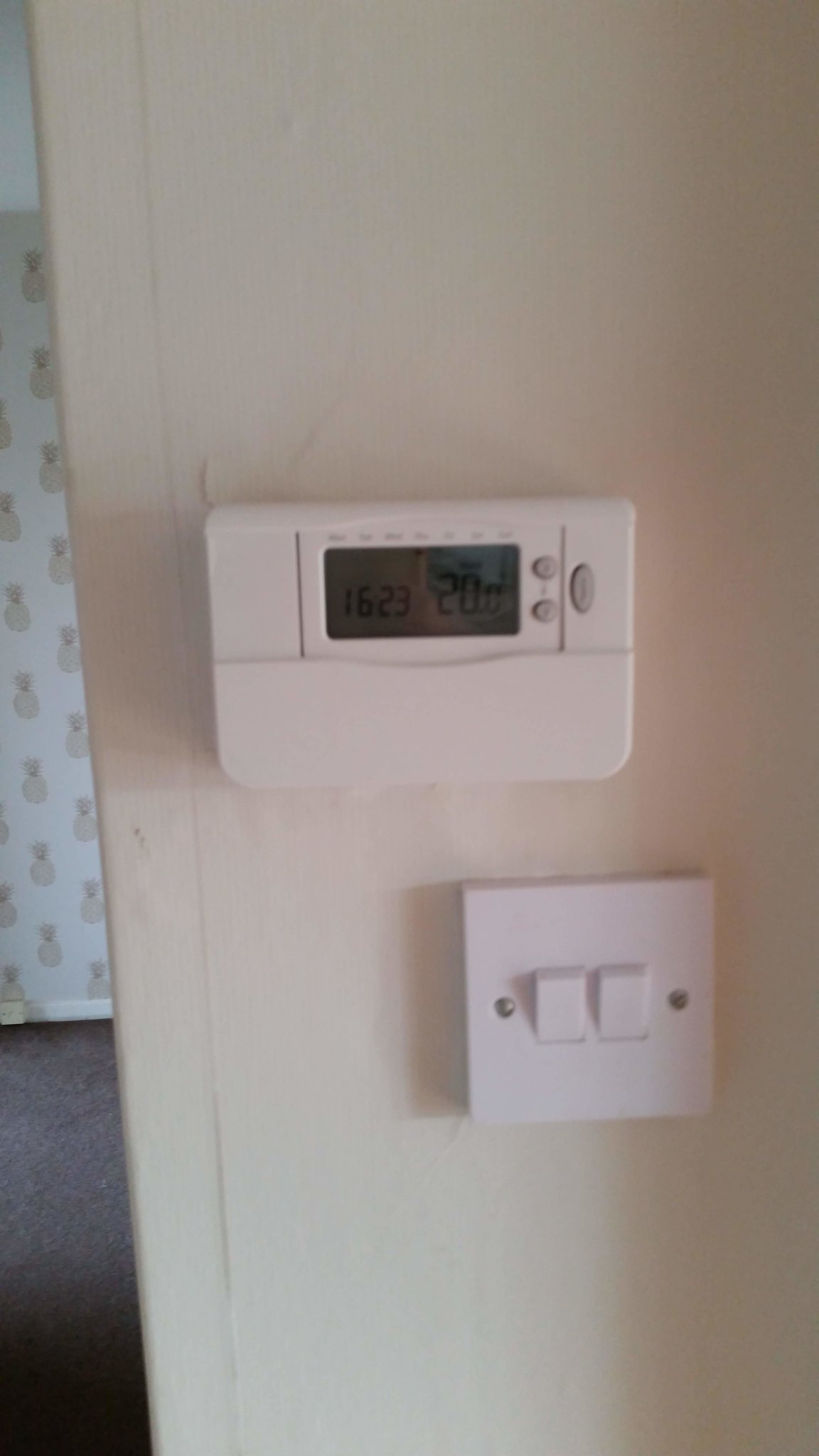The close-up image captures the corner of a room with a white wall as the focal point. On the left, a brown rug partially covers the floor, seamlessly transitioning into a wall adorned with a playful pineapple-patterned wallpaper. Prominently mounted on the white wall is a rectangular thermostat with rounded corners, crafted from white plastic. The thermostat screen displays the date "1623" along with the current temperature of "20 degrees." Directly beneath the thermostat, a square light switch is visible, featuring two toggles that both appear to be in the 'on' position. Soft shadows cast by the light switches add a subtle depth to the wall's smooth surface, enhancing the image’s overall detail.